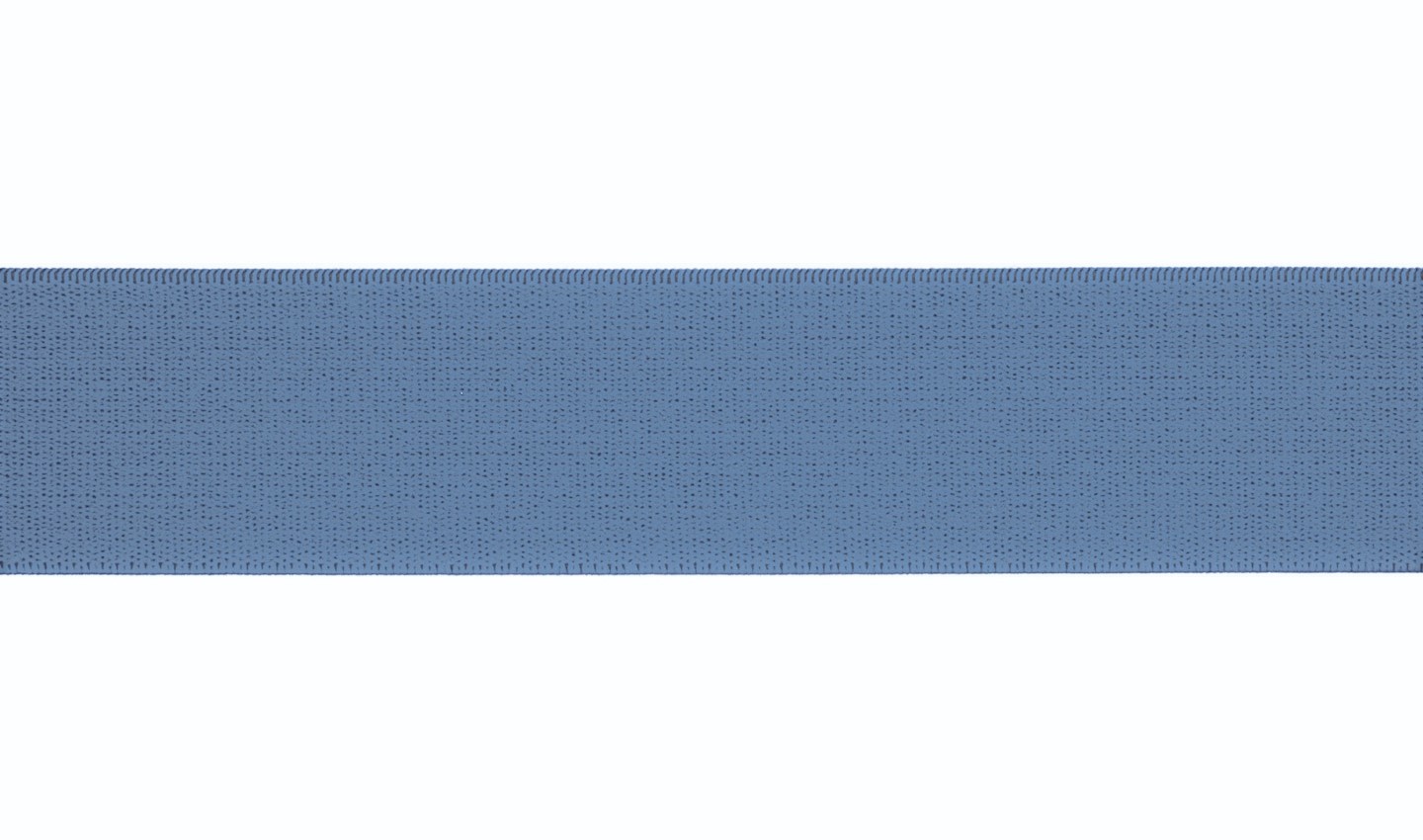The image showcases a thin blue strip of knitted fabric against a solid white void-like background, bordered on the top and bottom by white edges. The fabric strip, situated horizontally and centered across the image, resembles a textured ribbon or swatch, with its cool blue hue tinged with gray, emulating a steel-blue color. The left, right, and bottom edges of the strip are smooth, though it’s unclear if these are cut off from the photograph’s frame or intentionally designed that way. The top edge distinctly displays ridges, marking it as the outer end of the fabric. Scattered across the fabric, multiple small black holes punctuate the material, indicating areas with loose knots or incomplete knitting. The scene lacks any text or additional objects, emphasizing the simplicity and texture of the fabric strip against the off-white, egg-shell-colored backdrop.